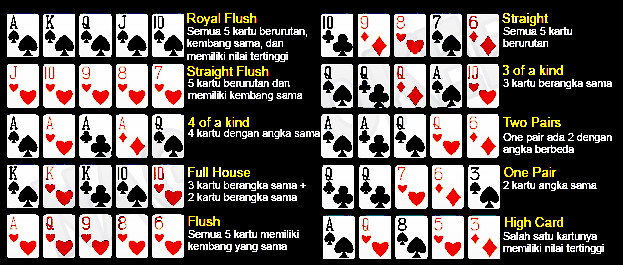In this vibrant and detailed color image, various winning poker hands are depicted in a gradient of arrangement from the highest-ranking to the lowest. At the top, there's the prestigious Royal Flush, showcasing the cards Ace of Spades, King of Spades, Queen of Spades, Jack of Spades, and Ten of Spades. Next, the Straight Flush is presented with the Jack of Hearts, Ten of Hearts, Nine of Hearts, Eight of Hearts, and Seven of Hearts. Following this, the Four of a Kind is displayed with four Aces (Spades, Hearts, Clubs, Diamonds) accompanied by the Queen of Spades. 

Continuing down, the Full House is portrayed with three Kings (Spades, Hearts, Clubs) alongside two Tens (Spades, Hearts). The Flush is exhibited with the Ace, Queen, Nine, Eight, and Six of Hearts. The Straight features the sequence Ten of Clubs, Nine of Diamonds, Eight of Hearts, Seven of Spades, and Six of Diamonds. Then, Three of a Kind is shown with three Queens (Spades, Clubs, Diamonds) alongside the Ace of Spades and Ten of Hearts.

Further down, Two Pairs is depicted with the Ace of Spades and Clubs, paired with the Queen of Spades and Hearts, accompanied by the Six of Diamonds. The One Pair hand features two Queen of Clubs accompanied by the Seven of Hearts, Six of Diamonds, and Three of Spades. Lastly, the High Card hand is presented with the Ace of Spades, Queen of Hearts, Eight of Spades, Five of Hearts, and Three of Diamonds. Each hand is meticulously arranged, providing a comprehensive visual guide to the hierarchy of poker hands.